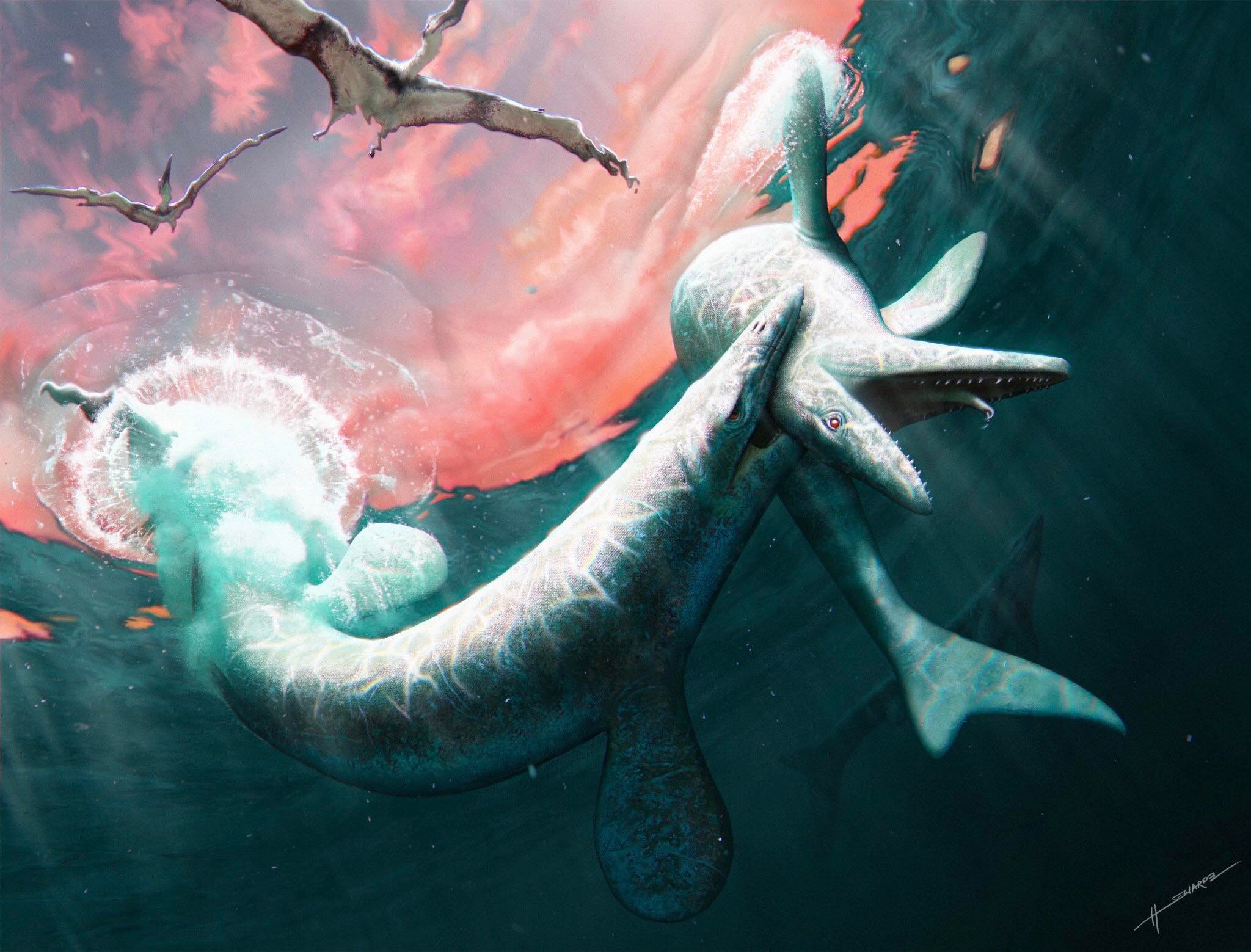This detailed painting captures the intensity of a dramatic underwater clash between two mosasaurs, their prehistoric whale-like bodies locked in a fierce battle. The scene is viewed from beneath the water's surface, providing a unique perspective that allows the viewer to see both the underwater struggle and the sky above. The water is clear, revealing a vibrant sky that transitions from a deep blue to a pinkish hue, dotted with puffy white clouds. Two pterodonts, or ancient winged reptiles, can be seen swooping towards the water, adding to the dynamic atmosphere. The mosasaur on the left has its teeth sunk into the neck of the other, pulling it downwards. The attacked mosasaur bends unnaturally at its midsection, with its tail pointed down and its head also facing downwards, a position exacerbated by the bite. The tail of the attacking mosasaur breaches the water surface, creating a splash and motion that highlights the violent encounter. At the bottom right of the painting, the artist's signature is visible, though it is difficult to decipher. This piece masterfully combines elements of ancient marine life and an action-packed moment, frozen in time with stunning detail.